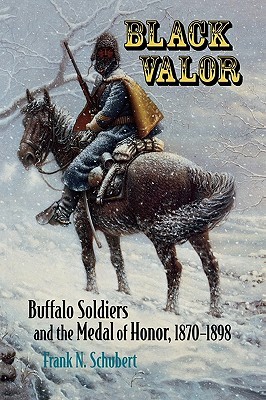The cover of the book "Black Valor" features an intricate design with a prominent block print title that transitions from gold to black. Beneath the title, the subtitle "Buffalo Soldiers and the Medal of Honor, 1870 to 1898" is printed in black, and at the very bottom, the author's name, Frank N. Schubert, is displayed in blue. The background is a wintry scene with falling snow, a snow-covered ground, and a leafless tree dusted with snow. Central to the image is a soldier sitting on a dark brown horse, both of them partially covered in snow. The soldier, clad in black clothing and a helmet, wears a gold cape that drapes over his frame, and holds a musket in his left hand. Additional details include a bedroll on the saddle, a sword hanging at his side, and reins nestled in the soldier’s hand. The horse has its head slightly bent, ice or snow visible on its coat, especially around its mane and tail. The scene exudes a sense of stillness and solemnity, perfectly capturing the historical and poignant atmosphere of the book’s subject matter.